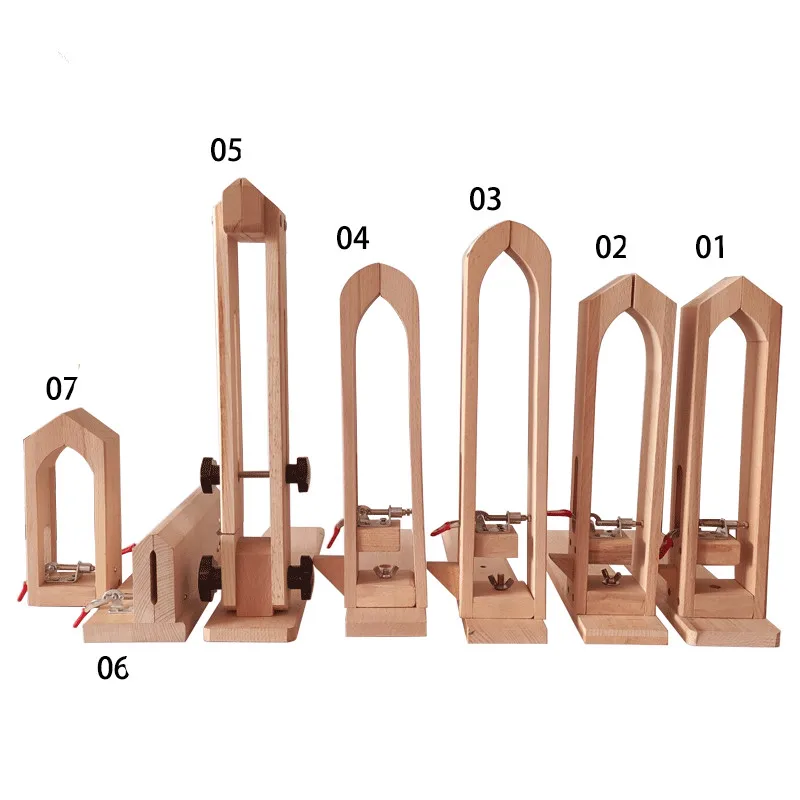The image depicts a series of seven wooden devices arranged from right to left against a white background. These devices, made of light brown wood, have been numbered 01 through 07 in black text, with the numbers starting from the right side. The structures are uniformly elongated with small rectangular bases and vary in height and shape at their tops. 

- Number 01 and 02, positioned on the right, have pointed tops. 
- Number 03 and 04 feature arched, rounded tops.
- Number 05 presents a mix of the previous styles.
- Number 06 is distinctively lying on its side, suggesting variability in placement.
- Number 07, on the far left, returns to having a pointed top.

Each device includes two pillars that support a U or V-shaped top and have a hole underneath. The pillars are mounted on a rectangular wooden base, connected by a metal nut and screw mechanism, indicating that these might be part of a woodworking project or a set of traps similar in build to mousetraps.